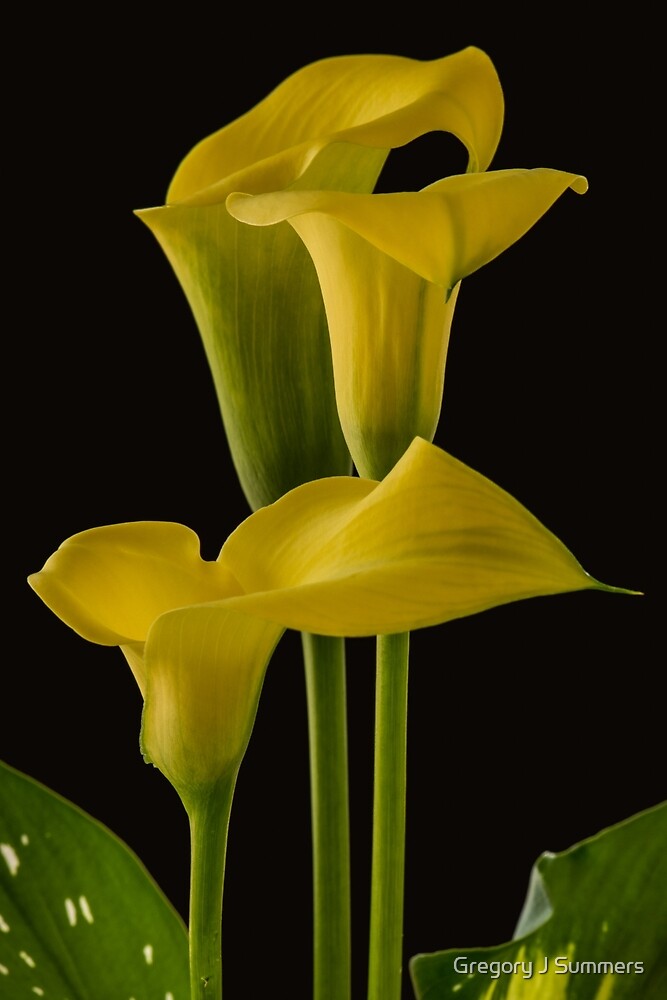The photograph, attributed to Gregory J. Summers as indicated by the small white font in the bottom right corner, showcases two yellow tulips set against a completely black background. The arrangement consists of three green stems, though only two tulips are prominently featured, one in full bloom and the other still closed, yet to fully blossom. The tulip petals are shaped like delicate pitchers with curved tops, adding to their graceful appearance. Flanking the flowers, partial views of green leaves are visible in the bottom left and right corners, providing a balanced framing. The overall simplicity and contrast of the black background emphasize the vibrant yellow and green hues of the tulips.